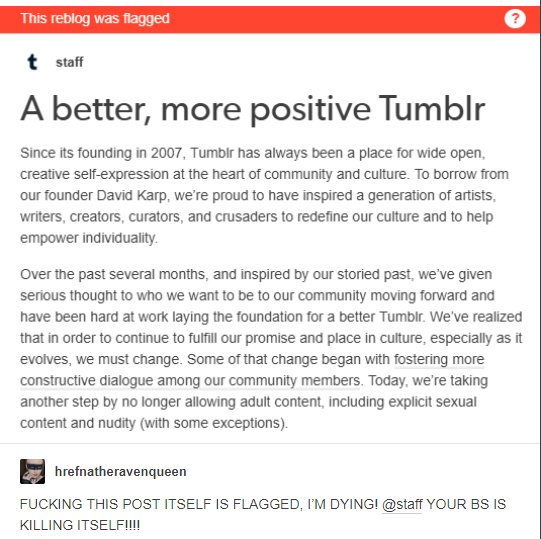This image is a screenshot of a Tumblr post featuring a blend of formal communication from Tumblr staff and a user comment. The background is white, with black text providing information. Across the top of the image, there is an orange banner with white text stating, "This Reblog was flagged." On the right-hand side of the banner, a white circle contains a question mark. The Tumblr "T" logo within a circle, followed by the word "staff," is prominently displayed.

The main blog post reads: 
"A better, more positive Tumblr. Since its founding in 2007, Tumblr has always been a place for wide-open creative self-expression at the heart of community and culture. To borrow from our founder, David Karp, we're proud to have inspired a generation of artists, writers, creators, curators, and crusaders to redefine our culture and to help empower individuality.

Over the past several months, and inspired by our storied past, we've given serious thought to who we want to be to our community moving forward and have been hard at work laying the foundation for a better Tumblr. We've realized that in order to continue to fulfill our promise and place in culture, especially as it evolves, we must change. Some of that change began with fostering more constructive dialogue among our community members. Today, we're taking another step by no longer allowing adult content, including explicit sexual content and nudity, with some exceptions."

Beneath this statement is a comment in all capital letters from a user, expressing frustration at the irony of the post being flagged: 
"FUCKING THIS POST ITSELF IS FLAGGED, I'M DYING, AT STAFF, YOUR BS IS KILLING ITSELF."